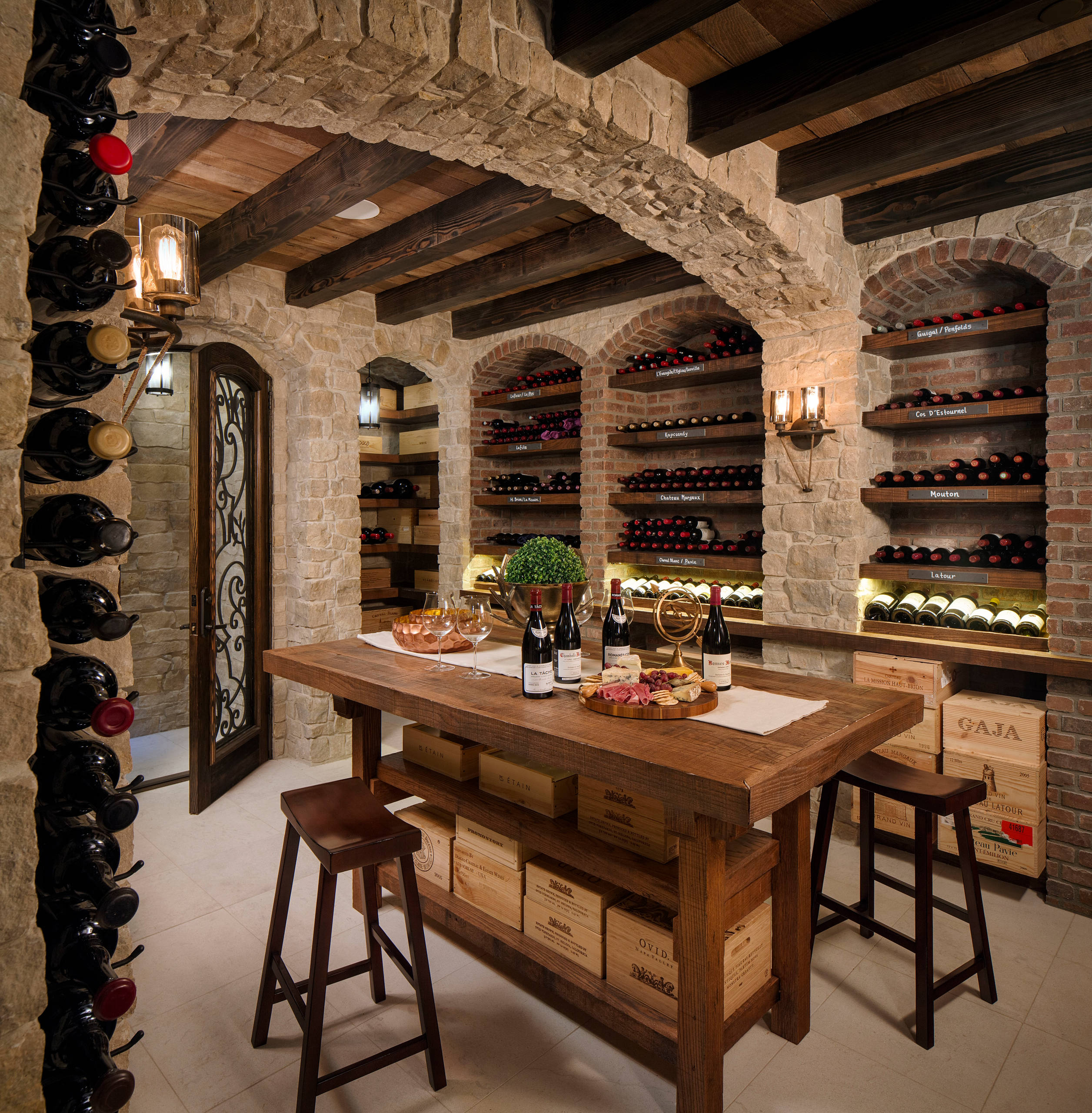The photograph showcases an elegant wine cellar, exuding an old-world charm reminiscent of an Italian setting. The room's stone brick walls and a ceiling adorned with massive wooden beams create a rustic yet inviting atmosphere. In the center of the cellar, a sturdy wooden table, covered with a white runner, is surrounded by two wooden stools on either side. Atop the table rest multiple bottles of red wine, primarily housed in dark bottles with red lids, alongside a houseplant and a snack plate, suggesting a setup for an intimate wine tasting session.

The foreground and background are lined with numerous shelves, meticulously stocked with an assortment of wines, many appearing in multiples of the same kind, hinting at a possible commercial space or store within the cellar. Additional boxes are stashed under the table, convenient for guests who might want to select and take home some bottles. The cellar's lighting is ambient, provided by strategically placed electric sconces, enhancing the cozy and relaxed atmosphere of the room. The space also features an archway made entirely of stone, which not only supports the ceiling but also serves as a striking visual element.

To the left, a line of wine bottles is prominently displayed, adding to the overall feel of a curated collection ready for tasting or purchase. The rear wall mirrors this aesthetic with its arched stone shelving laden with a variety of wine bottles. Adjacent to this is a small storeroom, visible through an open doorway, storing additional cases of wine. The floor is a lighter wood, possibly the subflooring from the above room, adding a touch of warmth to the otherwise earthy-toned space. This meticulous setting makes for a beautiful and clean environment ideal for a paid wine tasting experience in a classic, cool basement wine cellar.